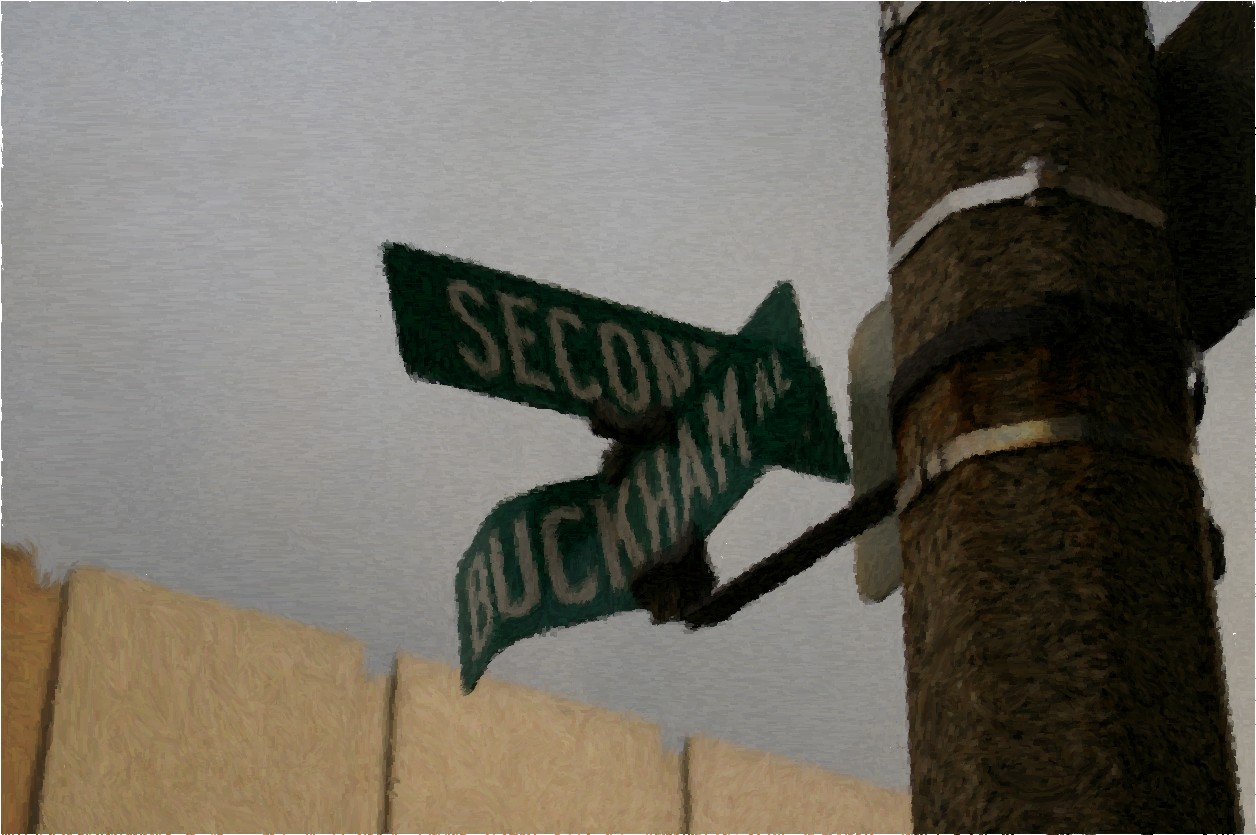The image depicts a digitally created or heavily edited photograph of a street corner where 2nd Street intersects with Buckham Alley. The street sign, depicting the street names in white text on green background, is attached to a large brown utility pole, which is secured with two silver metal bands, one at the top and one in the middle, and a black band between them. The sign appears damaged, being bent and crumpled, and is tilted at an odd angle. On the other side of the pole, part of another sign is visible. The closely cropped image includes a light brown wooden fence running diagonally across the bottom left corner. The sky in the background appears to be digitally altered and is nondescript, leaning towards a gray tone, contributing to the overall painterly effect of the image.